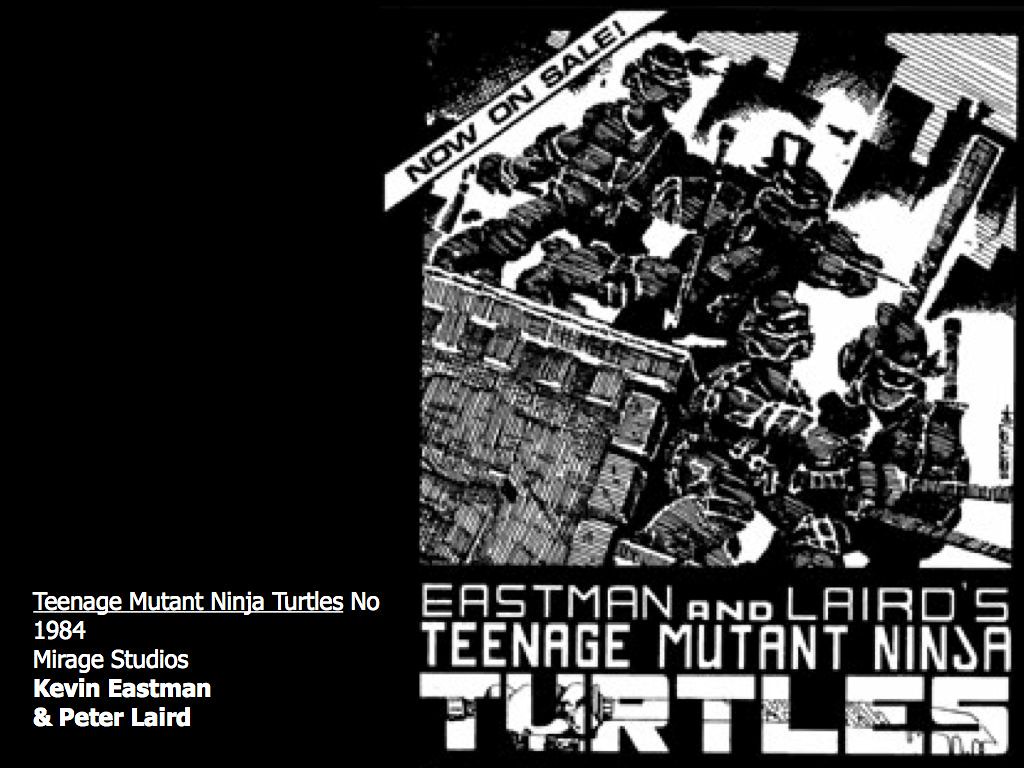This black-and-white image resembles an advertisement for the Teenage Mutant Ninja Turtles, set against a predominantly black background. The right two-thirds of the image is dominated by a dark, sketched drawing of all four Ninja Turtles; two are perched on a stone ledge while the other two stand at its base, partially obscured by the darkness. A faint cityscape with buildings can be discerned behind them. The image has a slightly tilted orientation. 

In the upper left corner, a white banner diagonally declares, "Now on Sale" in black print. Below the drawing, large white text states "Eastman and Laird's Teenage Mutant Ninja Turtles." The left third of the image is mostly black, but in the bottom left corner, white text reads: "Teenage Mutant Ninja Turtles N.O." followed underneath by "1984," "Mirage Studios," "Kevin Eastman," and "Peter Laird." The overall design is stark and primarily monochromatic, emphasizing the mysterious and gritty aesthetic of the Ninja Turtles.